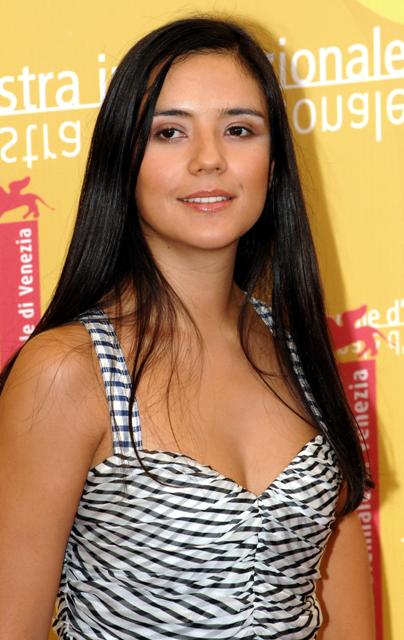This detailed photograph captures a young woman, possibly an actress in her mid-20s to early 30s, standing against a vibrant yellow promotional backdrop at what appears to be an international event or red carpet affair. Her slightly dark white skin and long, straight, black hair frame her face, which features minimal makeup and a slight smile, with her gaze directed off to the side. Her attire is a sleeveless top with thin straps, patterned in a textured black and white striped design reminiscent of zebra stripes. The promotional banner behind her is adorned with white text and is decorated with vertical red bars and a red-winged lion figure, with legible text "Di Venizia," suggesting an international or possibly Spanish-language event.